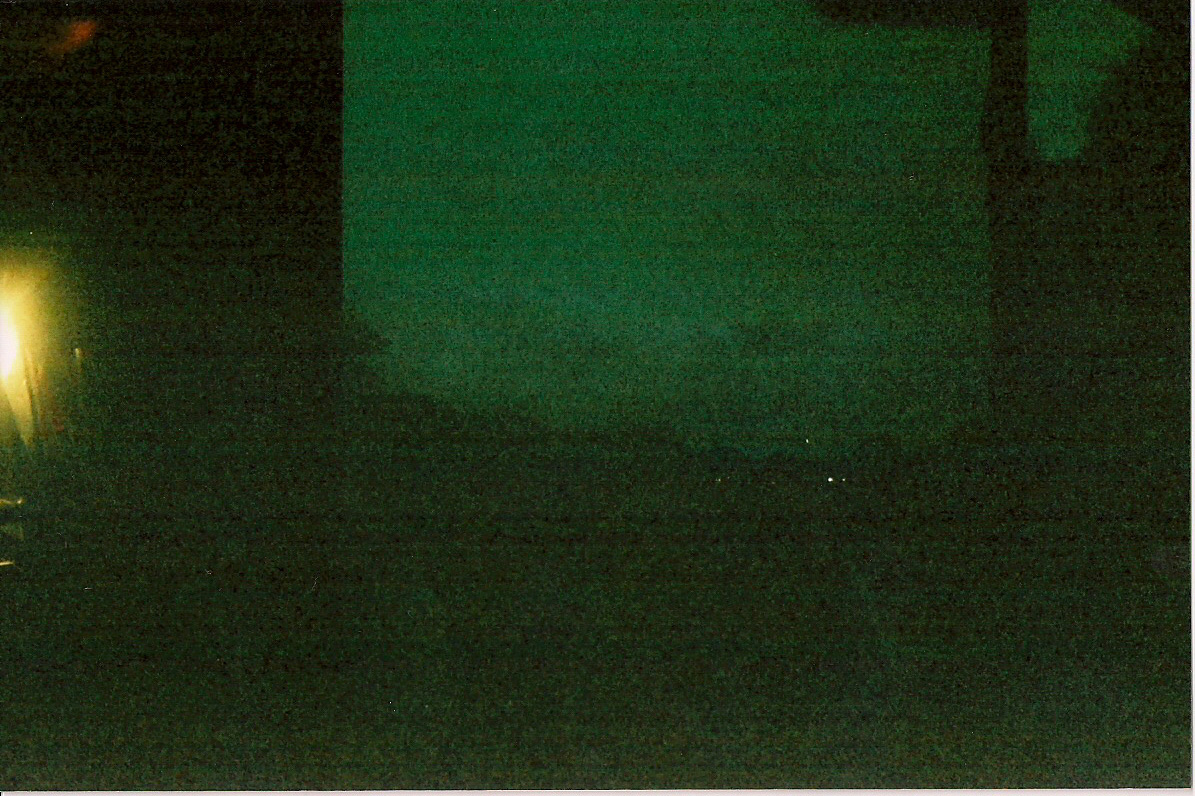This photograph is extremely dark and grainy, creating a blurry image with significant noise. The left side of the photo is almost entirely black, except for a small yellow light, possibly from a light fixture on a wall or building, located toward the far left edge. In the upper left corner, there's a tiny blotch of reddish-orange color.

The center of the image appears somewhat lighter, suggesting the presence of a doorway or window. Along the middle, there seems to be a horizon line, with faint indications of sky, possibly interspersed with distant lights, clouds, mountains, or trees. A curved shape is discernible in the center, indicating a division between the darker bottom and lighter top, implying the presence of the sky above.

As the image moves to the right, it becomes progressively darker. In the upper right corner, another lighter area is visible, which could be a view over part of a building into the same sky. The entire photograph is marked by horizontal bands of interference or low-resolution artifacts, characteristic of a very low-light photograph.